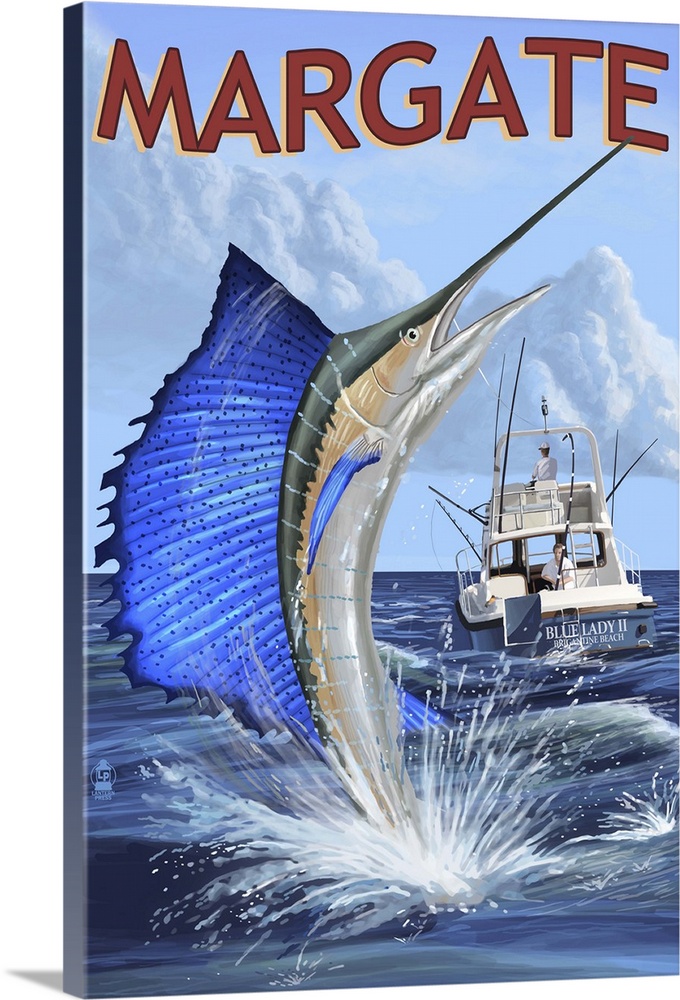This book cover mock-up features the title "Margate" in bold red lettering at the top, likely referencing the English town. The main image is a mid-century style painting, reminiscent of 1940s-1950s advertising art. Dominating the scene is a large, exotic fish, probably a swordfish or marlin, characterized by its sharp snout, blue fin with black dots along the top of its head, and prominent blue dorsal fin. The fish is dramatically emerging from the ocean, tail splashing in the water below a bright blue sky with scattered clouds. In the background is the rear view of a recreational fishing boat named the Blue Lady II, indicated by white letters on its hull. The boat, docked at an unspecified beach, has two occupants: one navigating and the other actively fishing with bent fishing rods indicating a catch. A small watermark in the bottom left corner reads "Lantern Press," featuring a lantern icon and text beneath it.